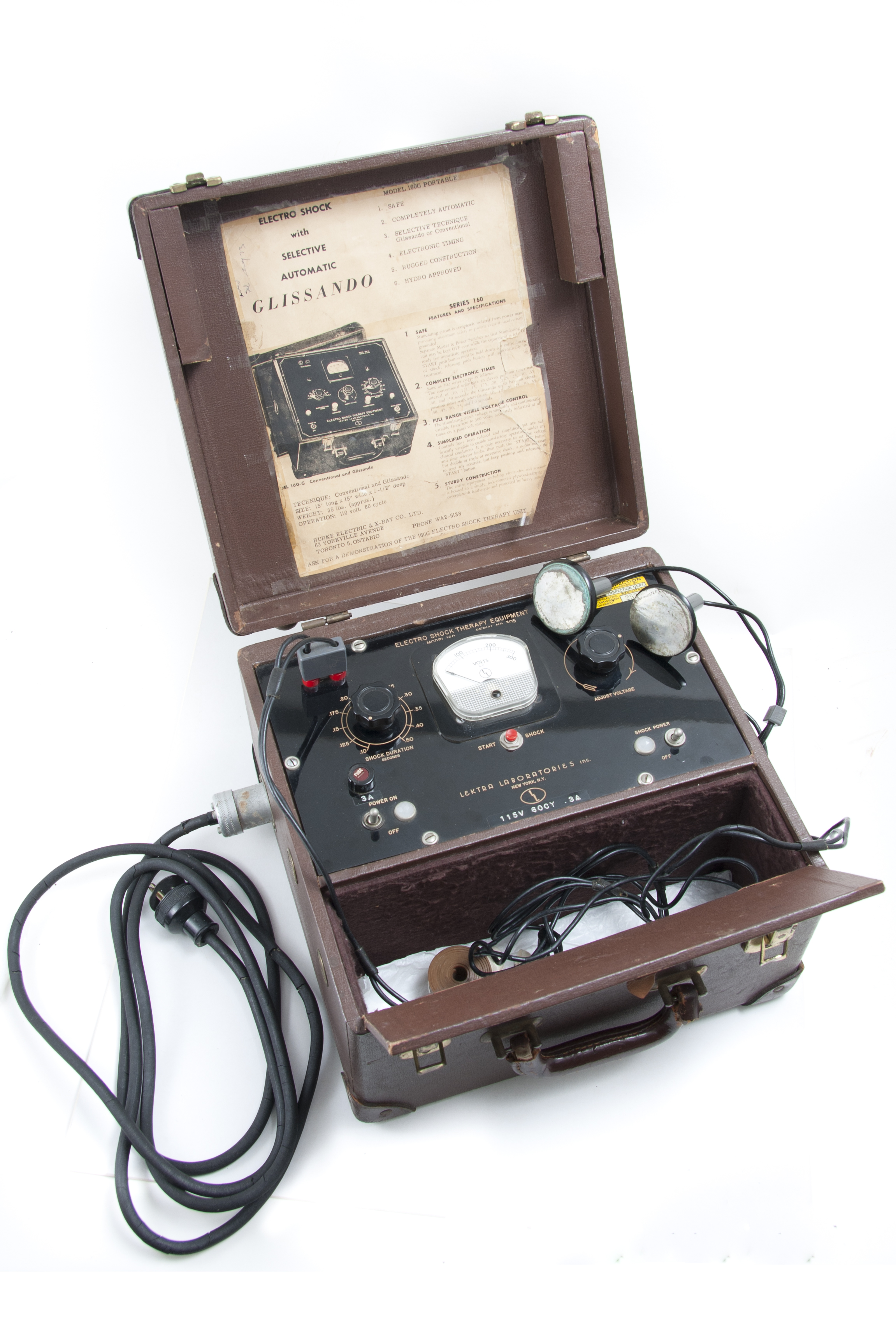In the image, set against an all-white backdrop, is a rectangular brown metal box with an open lid, revealing an intricate piece of machinery inside. The inside of the lid bears a tattered, cream-colored instruction paper, secured with tape, featuring the title "Electric Shock with Selective Automatic GLISSANDO," along with a detailed picture of the machine and smaller, less readable text. The box itself contains a black rectangular device equipped with dials, switches, a white gauge resembling a speedometer, and a distinctive red button. A silver plug is connected to one side of the box, with wires extending out in various directions. Additionally, there is a compartment within the box to store some of these wires. A prominent handle on the box suggests it is designed for portability.